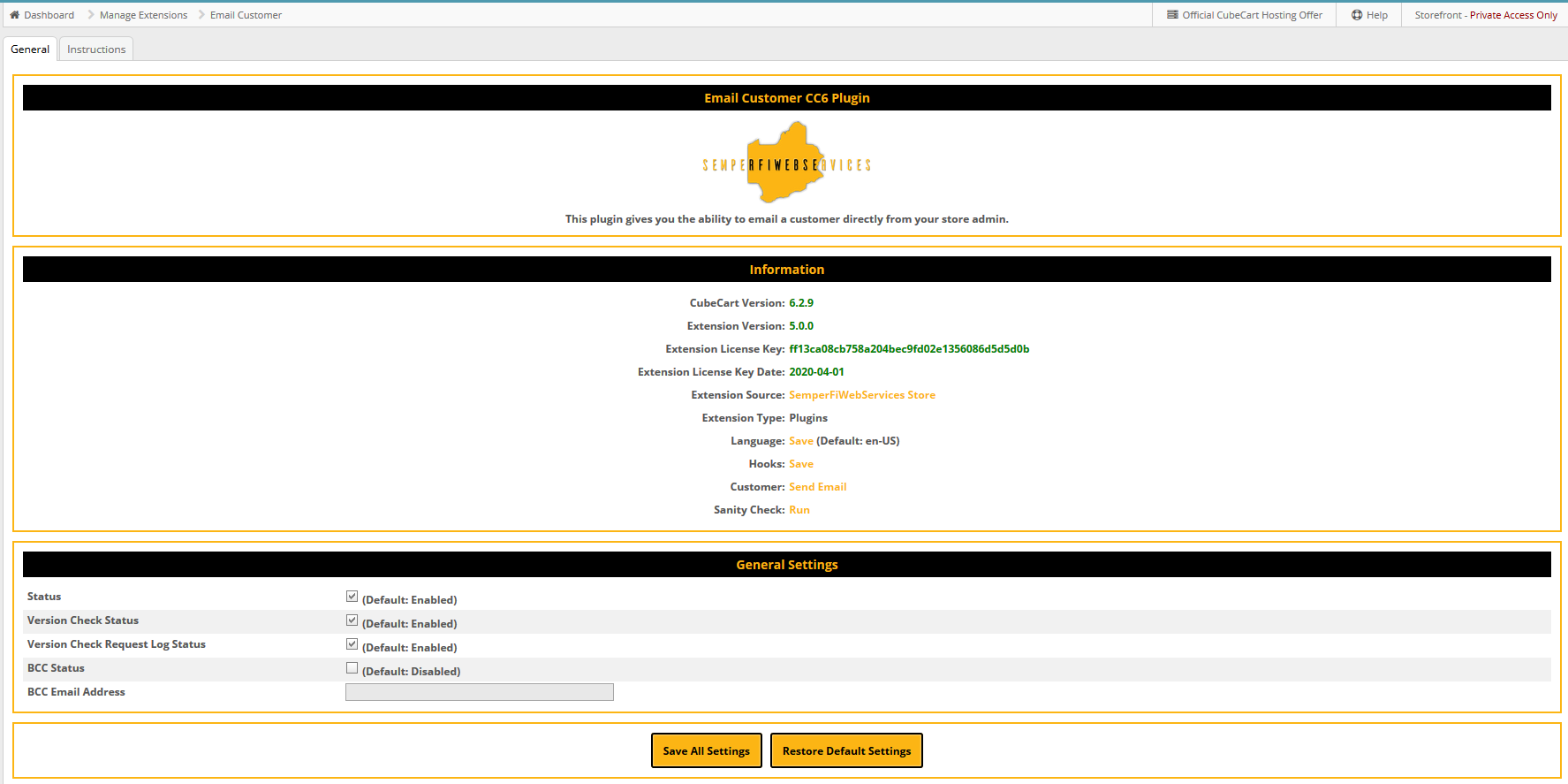Below is an enhanced and detailed caption for the given image:

---

The image showcases a partial web page interface, likely of a dashboard used for managing extensions and customer email functionalities. At the top, there are prominent tabs labeled "Manage," "Extensions," and "Email Customer." To the right of these tabs, some text is present along the top border, though it is unreadable.

Beneath the top border, the interface features two primary tabs: "General" and "Instructions," with the "General" tab currently selected. A black header bar with the text "Email Customer CC6 Plugin" caps the main content area of the page. Below this is a template section, which contains some unreadable text. However, it includes a description that reads, "This plugin gives you the ability to email a customer directly from your store admin."

Further down, there is another black section containing detailed plugin information: 

- Cue Cart Version
- Extension Version
- Extension License Key
- Key Date
- Extension Source
- Extension Type: Plugins
- Language Hooks
- Customer
- Security Check-In

Below this informational section is a "General Settings" area, highlighted by a black box. It lists the following settings alongside checkboxes:

- Status: ✅
- Version Check Status: ✅
- Version Check Request Log Status: ✅
- BCC Status: ✅
- BCC Email Address: ❌ (Default Enabled)

At the very bottom of the interface, within a white border, there are two buttons labeled "Save All Settings" and "Restore Default Settings."

---